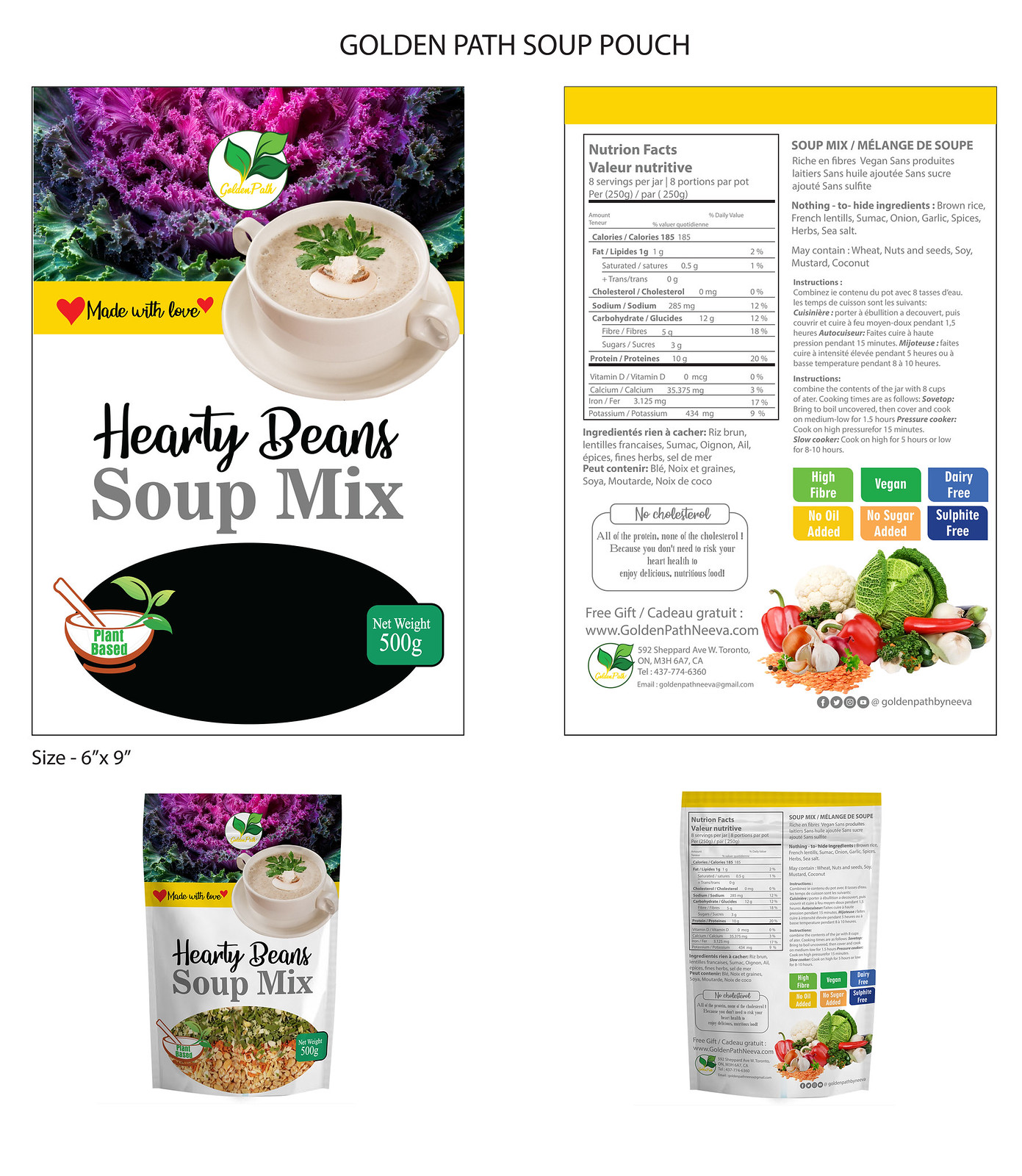The image is a detailed display of a hearty bean soup mix from Golden Path, showcasing four distinct elements. In the top left, there is an enlarged view measuring 6 inches by 9 inches of a generic poster for the soup mix, featuring a black oval shape with no image inside. Below this, there is a direct representation of the actual soup pouch, which includes a detailed picture within an oval frame. To the right of these images, there is an enlarged view of the nutritional facts label for the soup. Beneath the nutritional information, there is another representation of the soup pouch, showing its complete packaging design. Overall, the image effectively contrasts the generic poster and the actual product packaging, while providing a clear view of both the front and back of the soup pouch, as well as a detailed look at the nutritional information.